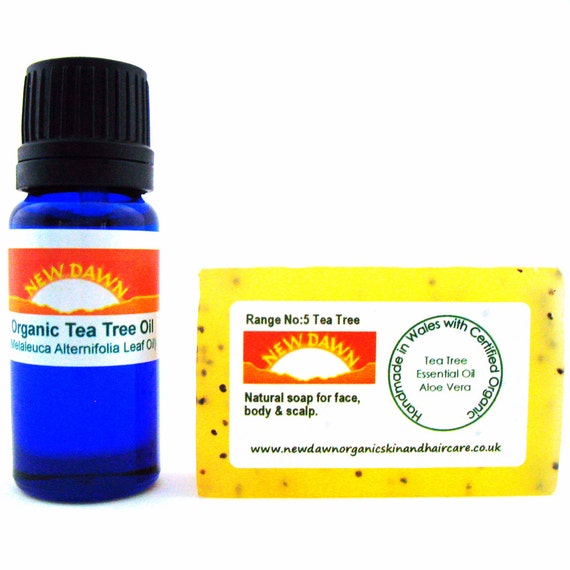The photograph depicts a collection of New Dawn Organic Tea Tree Oil products against a white backdrop. On the left, there's a small, blue see-through glass bottle of tea tree oil with a ridged black cap for easy opening. The bottle's label features a sunset logo with "New Dawn" in yellow letters curving around the image, set against orange and red hues. The label reads "Organic Tea Tree Oil" and "Melaleuca alternifolia leaf oil" in parentheses. To the right of the oil, there's a yellow, speckled bar of handmade soap labeled "Range No. 5 Tea Tree". The soap, designed for face, body, and scalp, carries the same New Dawn logo as the oil. Additionally, the soap's label mentions it contains tea tree essential oil and aloe vera and includes a "Handmade in Wales and Certified Organic" sticker. Both products feature the website www.newdawnorganicskinandhaircare.co.uk printed at the bottom of their labels.